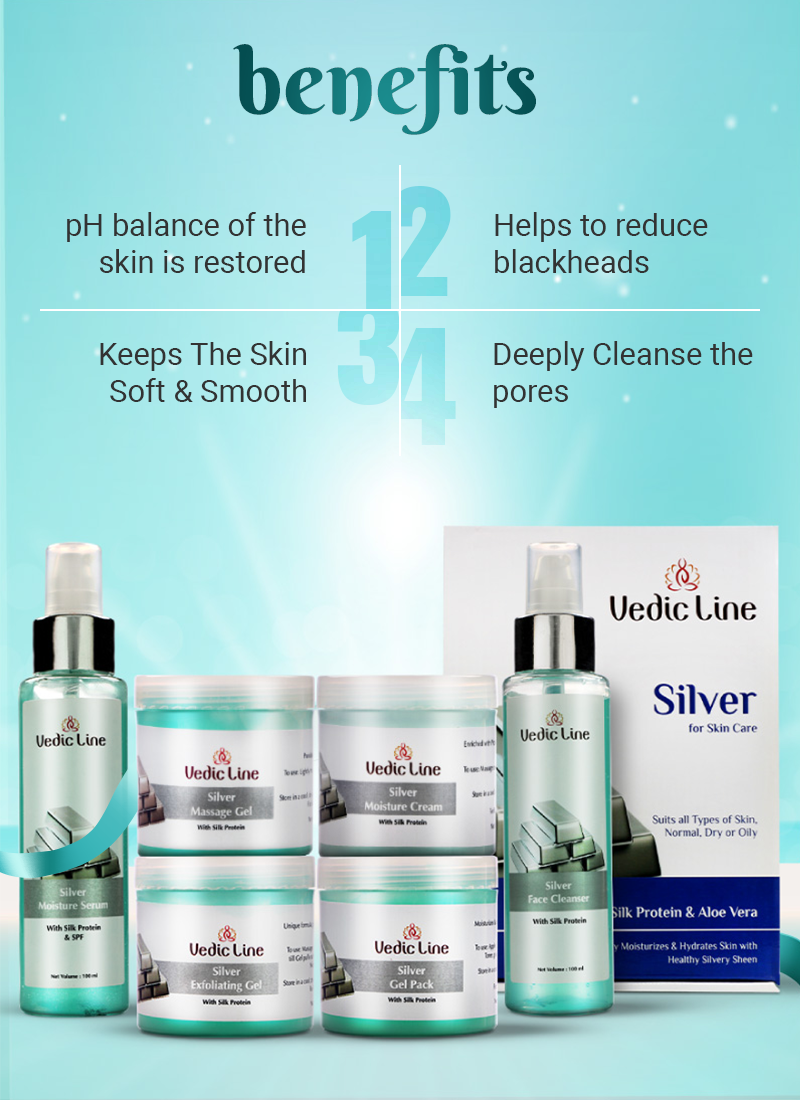This is an advertisement for a skincare line called Vedic Line. The background of the poster transitions from a bluish-green at the top to a light blue towards the center, with a prominent light or sunburst effect illuminating the products. At the top of the poster, "Benefits" is written in blue letters, followed by a detailed list in four sections: "1) pH balance of the skin is restored, 2) Helps to reduce blackheads, 3) Keeps the skin soft and smooth, 4) Deeply cleanses the pores." The lower half of the poster showcases the skincare products, which include two spray bottles and four jars or tubs with seafoam green and white labels. Each product prominently features the Vedic Line logo. A white card stands behind the spray bottle on the right, indicating the product suits all skin types—normal, dry, and oily—with additional mentions of ingredients like silk protein and aloe vera in blue boxes. No models or people are present, ensuring an exclusive focus on the Vedic Line products and their highlighted benefits.